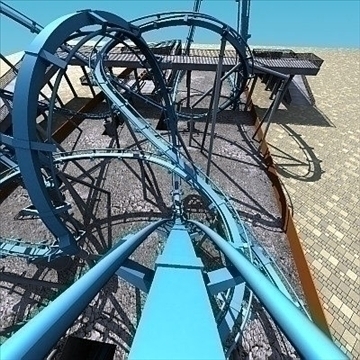This image provides a first-person perspective from the front cart of a roller coaster at an amusement park, capturing the thrilling descent down a set of light blue roller coaster tracks. The background features a clear blue sky, contributing to a bright daytime setting. The ground beneath the track varies in color, displaying areas of gray cement and patches of light tan and brown. On either side of the tracks, there are maintenance platforms, indicating where staff might work on the coaster. The photo, seemingly taken in motion, shows looping structures in the background, emphasizing the dynamic and adventurous nature of the scene. The roller coaster is well-centered in the image, with additional detailing of gray flooring to the right and a section of tan in the left background, reinforcing the outdoor amusement park context.